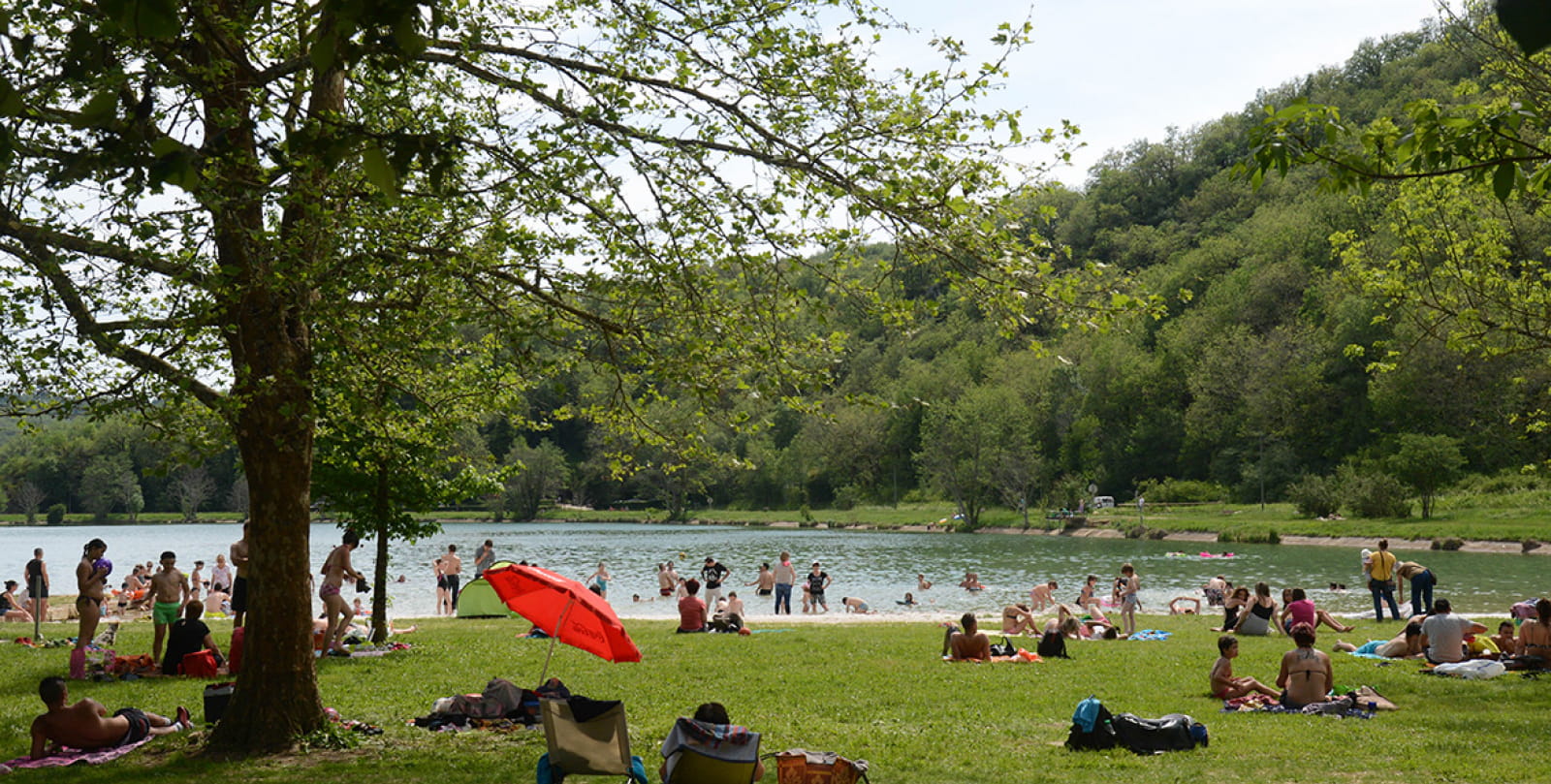The photo captures a lively lakeside scene on a mostly clear day, featuring around 40 to 50 people enjoying various activities. In the foreground on the left, a large green tree provides shade to individuals lounging on towels. The lake, with its dark green water, stretches across the middle of the image, surrounded by plush greenery and hills densely packed with trees. People in swimsuits are scattered throughout the area: some are swimming, others are gathered near the sandy shore, and several are sitting on chairs or blankets, including a person under a red umbrella. Children are seen playing in the sand, and many groups appear to be deeply engaged in conversation. Tree branches frame the scene from the top right, adding to the picture's natural ambiance.